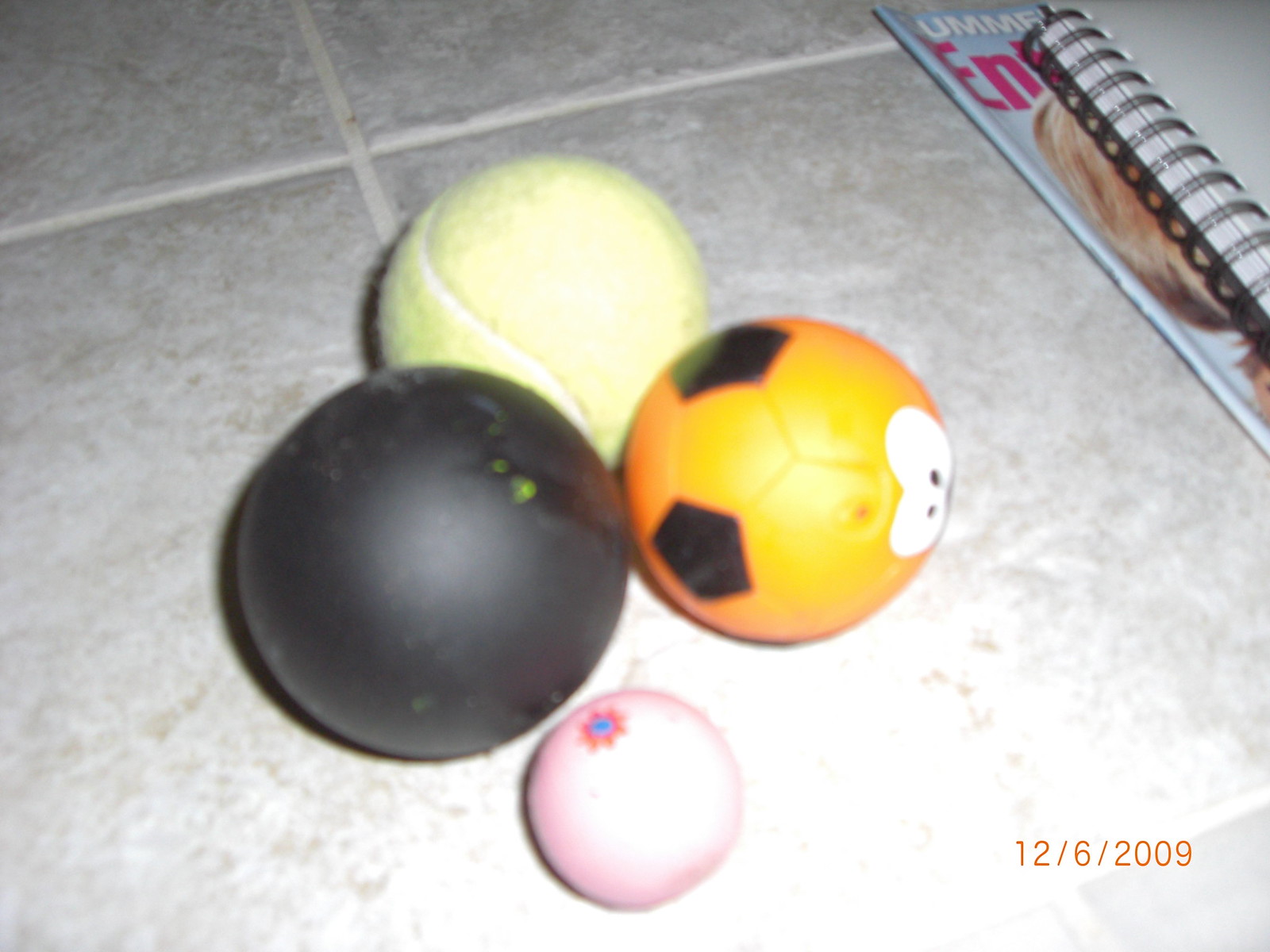Captured on December 6, 2009, the image features a close-up of four balls arranged in a diamond shape on a light grayish-tan tiled surface. The distinct balls include a yellowish tennis ball, a solid black ball, a tiny pink ball with a small blue speck and a red starburst around it, and an orange ball with black hexagons and white and black eyes. Additionally, on the upper right side, part of a magazine with the letters "U-M-M-E" and a spiral notebook on top can be seen.